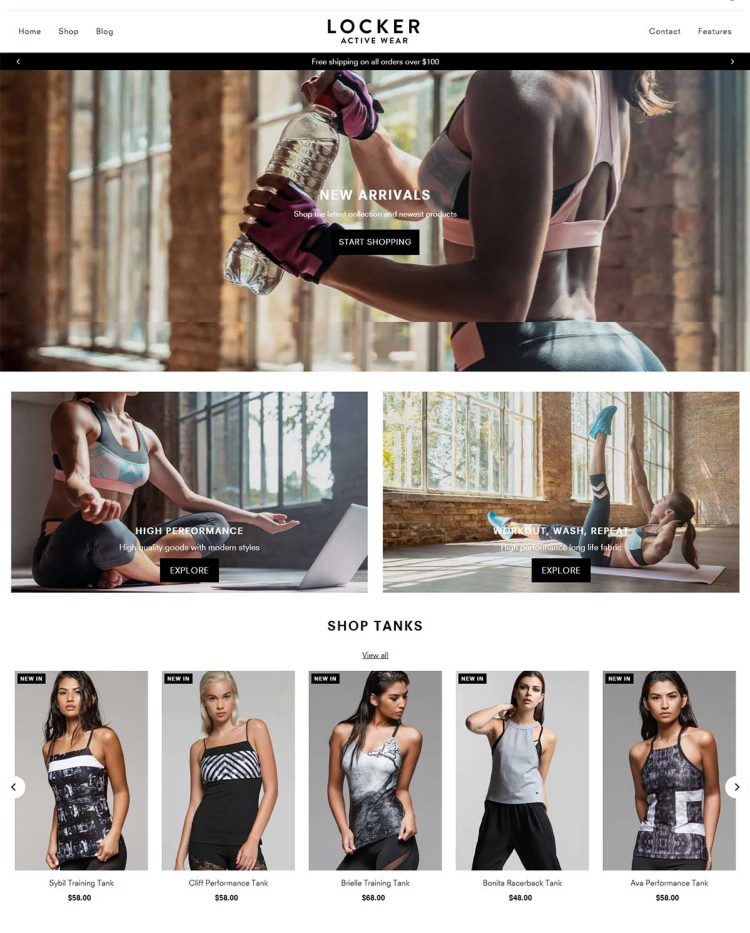The image has a slightly vertical rectangular frame, presenting a structured and visually engaging layout from a website screenshot. At the top, on a white background, are navigation links: "Home," "Shop," and "Blog" positioned on the left, "Locker Activewear" boldly centered, and "Contact" and "Features" on the right.

Just below the navigation bar, several images occupy the frame. The top image spans the entire width of the frame, showing a segment from the shoulder to the waist of a woman dressed in sports attire, holding a water bottle. Overlaying this image are the words "New Arrivals" with a "Start Shopping" button presented prominently.

Beneath this, two horizontally rectangular images are arranged side-by-side. The left image displays a woman in a cross-legged position, visible only from the neck down. Text overlaying this image reads "High Performance" with an accompanying "Explore" button. The right image shows a woman lying on her back, her left leg raised and her right arm reaching toward her left foot, captioned with "Workout, Wash, Repeat" alongside an "Explore" button.

Finally, at the bottom center of the frame is the caption "Shop Tanks," accompanied by five side-by-side images of different models wearing tank tops, showcasing the variety of styles available.